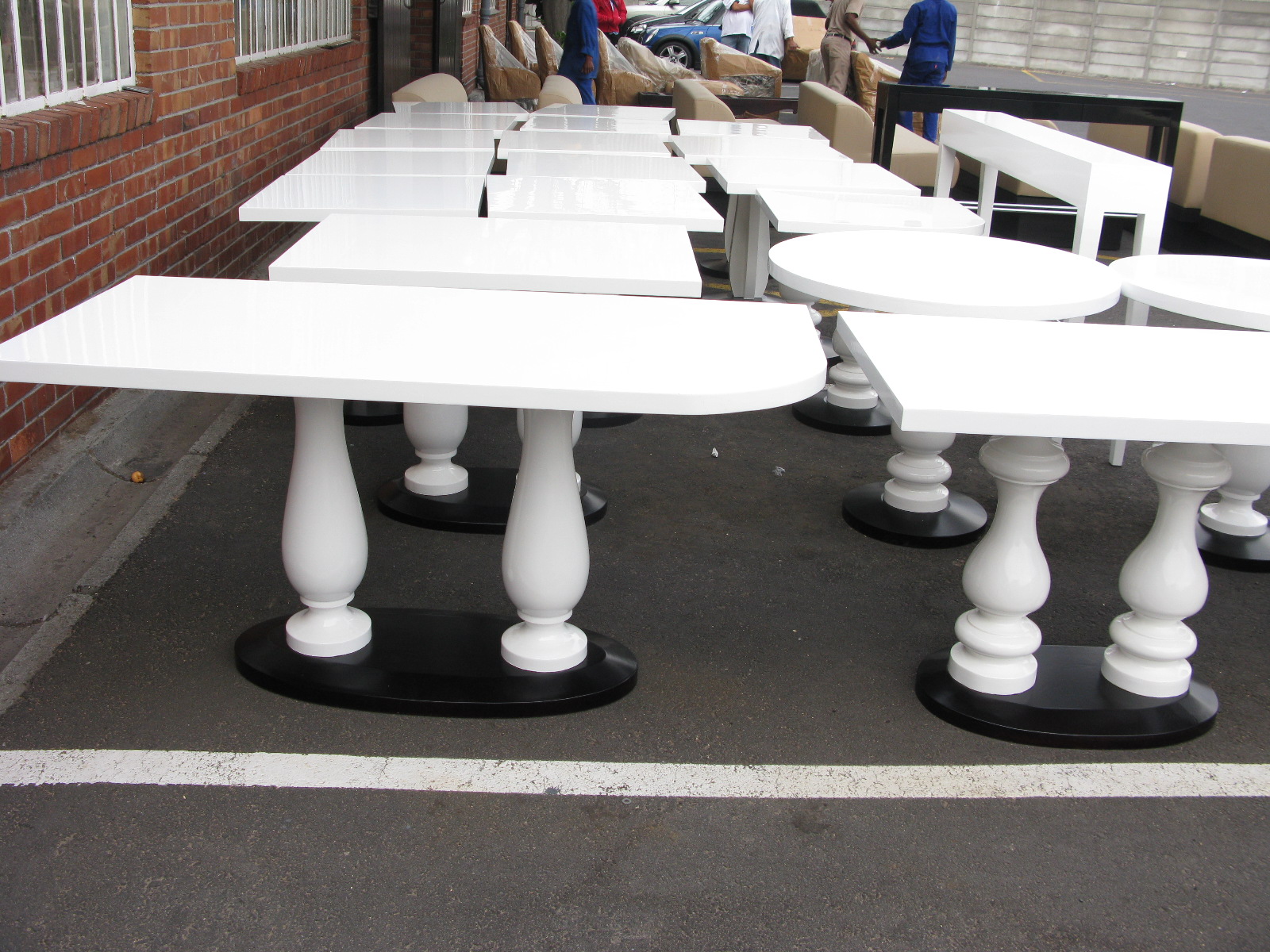The photograph captures an outdoor furniture display, likely set up in a parking lot. The scene is dominated by an array of white tables of various shapes and sizes, featuring both rectangular and circular tops. Each table rests on ornate, lathed pedestal bases reminiscent of chess pieces or stair banisters, which are thick and intricately designed. These white pedestals sit atop black, flat circular bases, adding to their sturdy appearance.

In the foreground, there is a uniquely shaped table with a rounded corner, supported by two pedestal bases. The background features smaller square tables and a brown table interspersed with beige chairs, hinting at a broader range of furniture on display. The setting includes a red brick wall on the left, punctuated by white-framed windows with bars cutting off midway.

To the right, the pavement extends, marked by white lines typical of parking spaces. Distant figures can be seen, involved in various activities—some appear to be moving furniture or engaging in business dealings, while others stand near cars. Wrappings on some chairs suggest they are part of a setup process. A transparent white wall in the far background further encloses the area, adding a layer of ambiguity to the open-air setting, possibly indicating a partially covered display area.